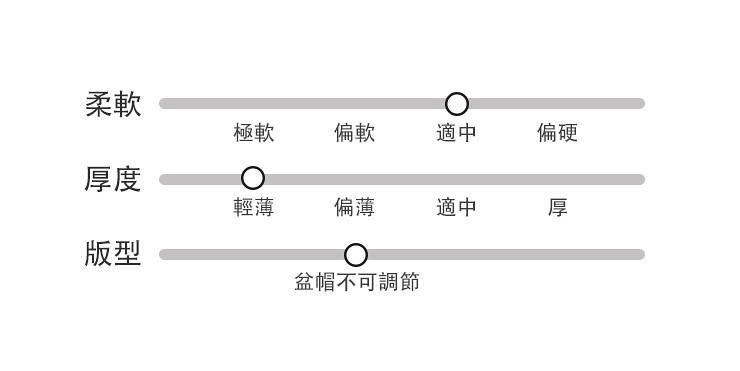The image displays a simple yet detailed interface, likely part of a survey or adjustment feature, featuring three horizontally aligned sliding scales. Each scale is gray and equipped with a small white circle, positioned as if someone has interacted and dragged it along the scale. Each scale is accompanied by characters, likely in Chinese or Japanese, which appear both to the left of each line in large black print and beneath each line in smaller grayish-blue print. The first two sliding scales have four selectable options, with the circles indicating different positions along these scales. The third scale differs, presenting only a single option where the circle rests. The sliding scales are uniformly spaced, with approximately a centimeter between each, and are identical in length. This structured layout suggests a methodical approach to setting levels or expressing degrees of agreement, with particular attention to detail in the multilingual labels and the precise arrangement of elements on the image.